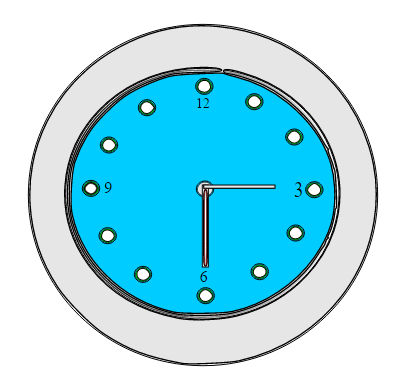This image showcases a meticulously crafted digital drawing or printout of a clock. The clock's design features a black outer circle serving as a bold border. Inside this border, there is a grey, hollow ring reminiscent of a doughnut, adding a layered frame effect to the visual. Enclosed within the grey ring is another black circular line, creating a defined outer edge for the clock face. The clock face itself is a very light blue, offering a subtle and calming background. 

The hours 12, 3, 6, and 9 are distinctly marked, with the other numbers omitted, giving the clock a minimalist yet structured appearance. Above the 12 is a prominent open white circle, which resembles a white dot encircled by a black ring. Identical markings repeat uniformly around the clock's face, creating a pattern of 12 such circles, aligning perfectly with each hour. The clock shows the time is 3:30, with the minute and hour hands positioned accordingly, forming a visually balanced and precise depiction of time.